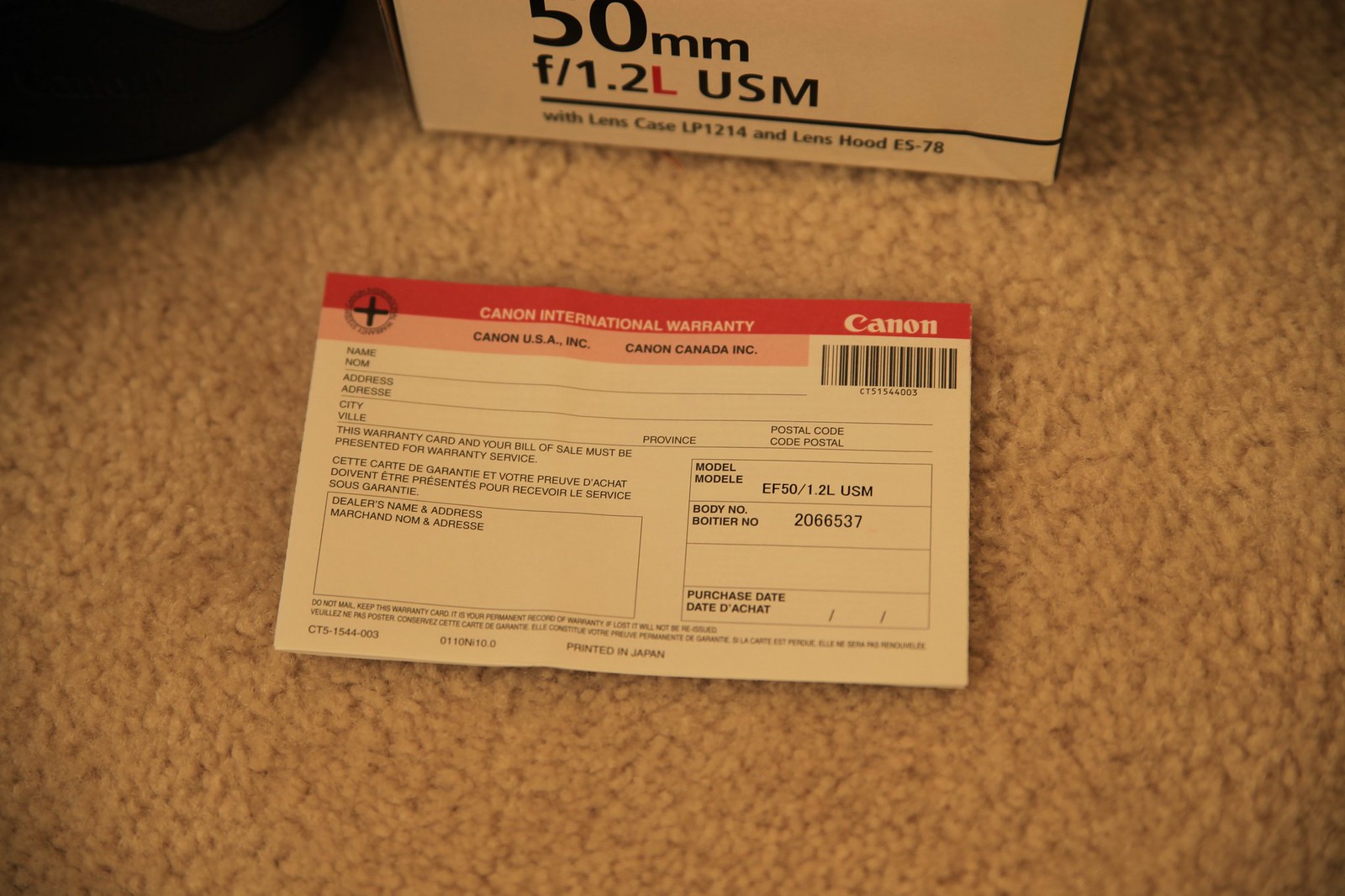This color photograph captures a warranty card resting on a brown carpet. Prominently positioned in the background is a white box labeled with "50mm f/1.2L USM," which includes additional details about the contents—"Lens Case LP1214" and "Lens Hood ES-78."  

The warranty card features a striking red banner at the top that displays "Canon International Warranty," alongside the logos and names of "Canon," "Canon USA Inc.," and "Canon Canada Inc." Additionally, a barcode marked as "CT51544003" is printed near the top. 

The card itself contains an unfilled form with fields for personal details: "Name," "Address," "City," "Province," and "Postal Code." There's also a notice emphasizing that the warranty card and bill of sale must be presented for warranty service, alongside fields for the dealer's name and address. The dealer's section is partially completed with "Model: EF50-1.2L USM" and "Body Number: 2066537," but the "Purchase Date" remains blank. 

At the bottom of the card, important instructions advise the user, "Do not mail. Keep this warranty card. It is your permanent record of warranty. If lost, it will not be reissued." Beneath the English text, all information is translated into French. 

The photograph meticulously documents both the primary language and its French translation, capturing every nuanced detail of the warranty card's content and the meticulously organized scene.